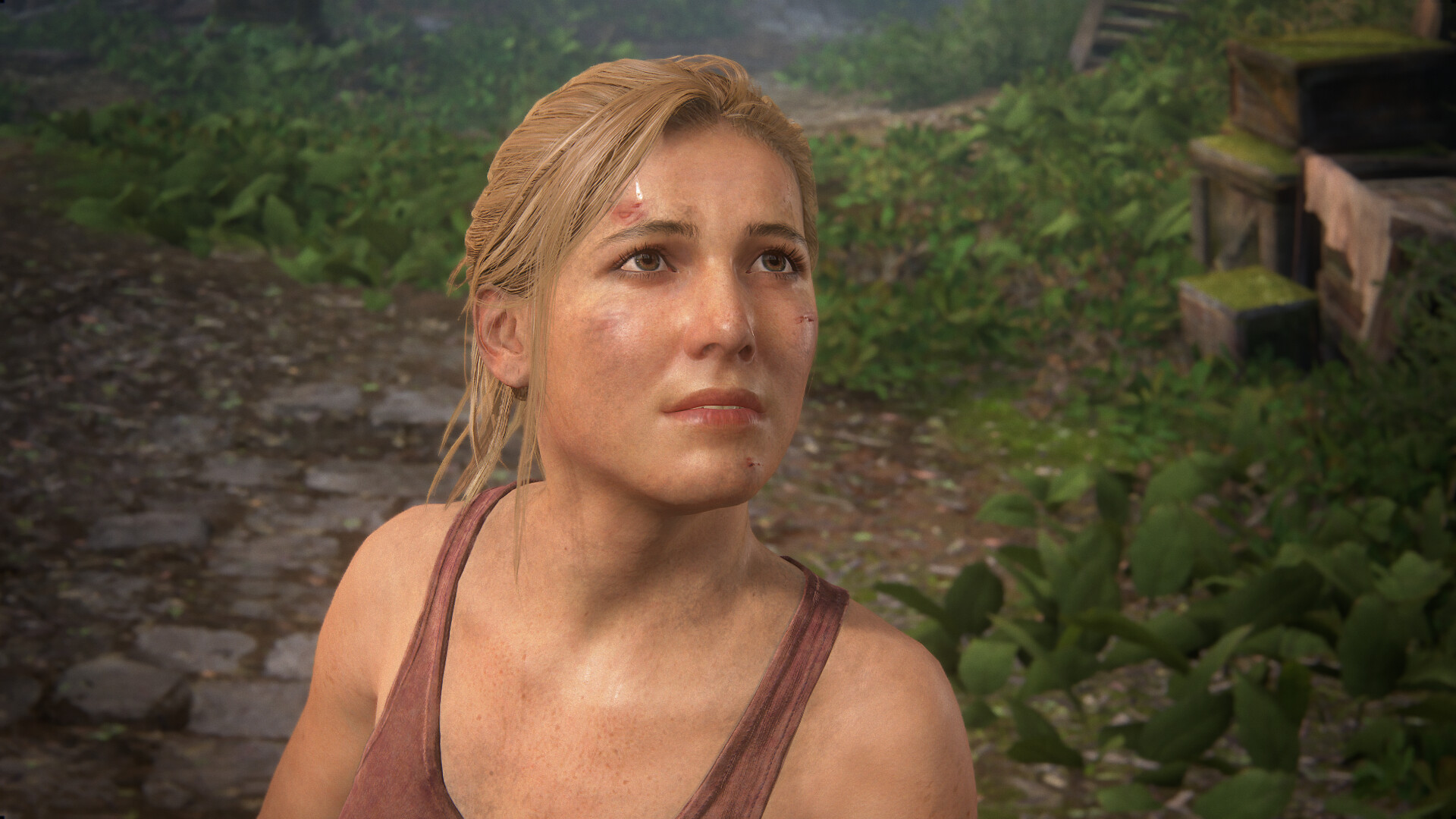A highly detailed close-up of a female video game character rendered with impressive CGI realism. Her blonde hair is pulled back, with a few loose strands framing her face. She has noticeable bruises on her cheeks and a scrape on her forehead just above her left eye. Her expression is one of determination as she gazes upward to the right. She is clad in a maroon or purple tank top and appears to be perspiring, adding to the intense atmosphere of the scene. The background depicts a rugged jungle environment with a broken concrete pathway visible to her left. The area is overgrown with lush greenery sprawled across the bottom right, top left, and top right of the image. Additionally, there are crates beside a small concrete divider wall on the ground, which is also covered with patches of vegetation, amplifying the sense of an abandoned, untamed setting.